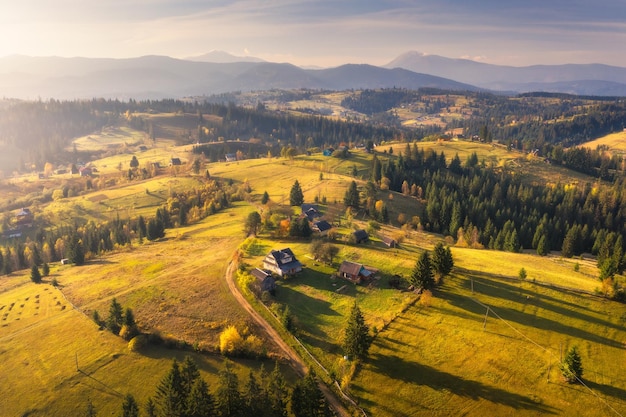The image is a detailed landscape photograph captured from a high vantage point, possibly by a drone or helicopter. It provides a bird's eye view of a largely rural area characterized by sprawling green fields, patches of dense forest, and a scattering of small, rural houses. The vibrant green of the grass is illuminated brightly by the sunlight, which is positioned low in the sky, casting long shadows across the terrain. In the middle of the image, tiny houses and buildings are visible, surrounded by green fields that stretch out to the left and right. Towards the top of the image, the land transitions into rolling hills adorned with tall pine and fir trees. These hills are interspersed with fields and flatlands, suggesting areas of farmland. In the far distance, blue mountains rise against a bluish-gray sky, which fades from lighter shades on the left to darker tones on the right. This composition beautifully captures the vastness and natural beauty of the rural landscape.